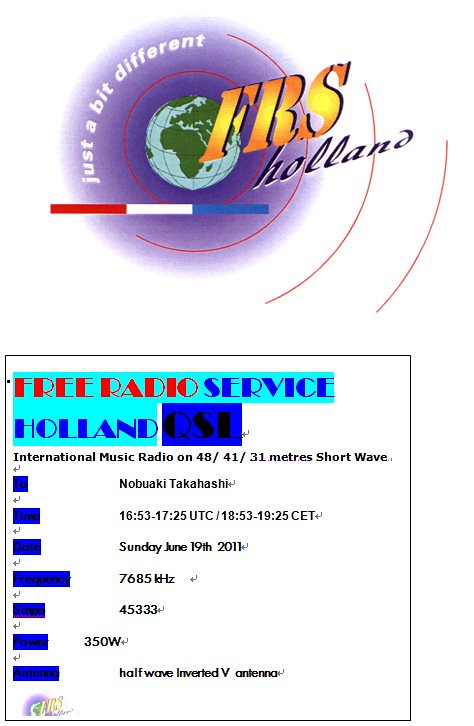The image is an advertisement for the Free Radio Service (FRS) Holland radio station. It is divided into two main sections. The top portion features a globe at the center encircled by a purple sphere and a semicircle, with a red line spiraling around it. Around the purple area, in white text, it says "Just a Bit Different." Shooting out of the globe are the gold letters "FRS," followed by "Holland" in black script. Below this is a horizontal bar in the Dutch national colors—red, white, and blue.

The lower section is a square with detailed informational text. It announces "Free Radio Service Holland QSL," along with additional descriptors such as "International Music Radio on 48/41/31 meters shortwave." The broadcast details include the name Nobuaki Takahashi, day and time of the broadcast as Sunday, June 19th, 2011, from 1653-1725 UTC (1853 to 1925 CET), on the frequency 7,685 kilohertz, with a signal report of 45,333. It indicates that the broadcast is transmitted at 350 watts using a half-wave inverted V antenna. The background of this section is white.